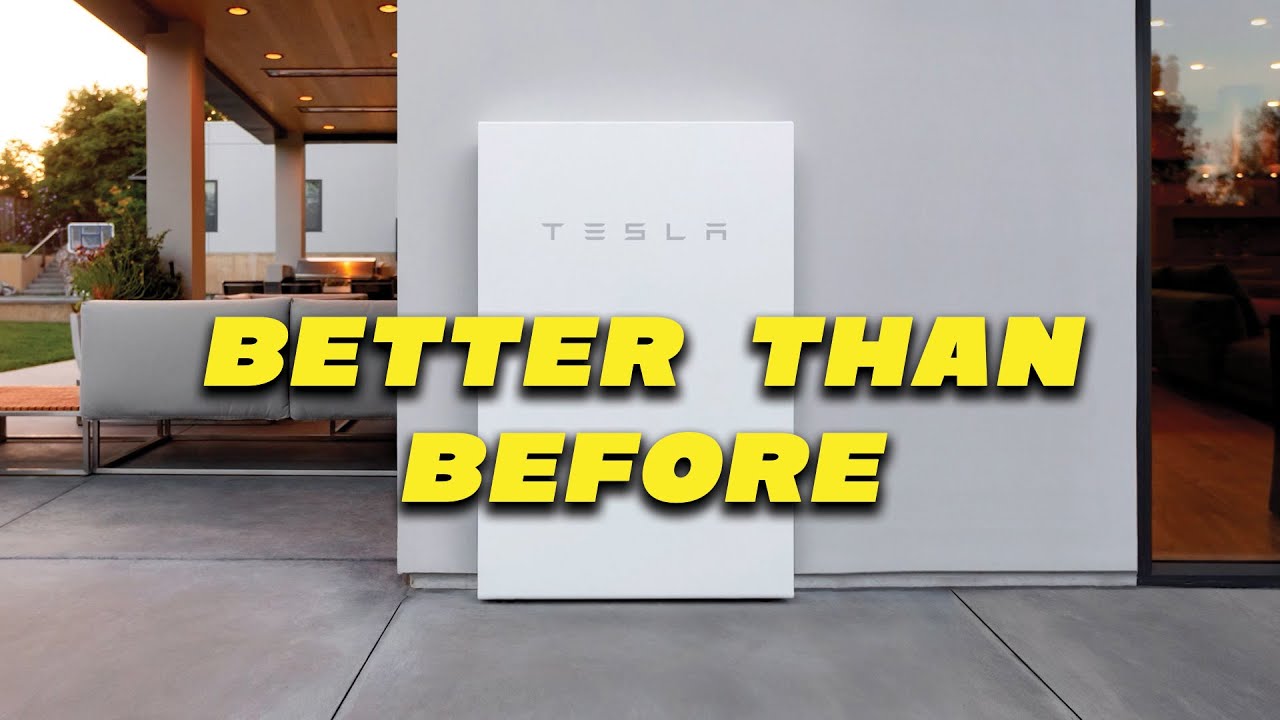In this image, a vibrant text message "Better Than Before" dominates the center, written in bold yellow letters with a distinctive black shadow effect. This striking text overlays a picturesque scene capturing a serene veranda. Propped against a grey building wall is a sleek white Tesla Powerwall, marked with the brand name "Tesla" in subtle grey. 

To the right, the building features a glass door framed in black. The flooring consists of large grey tiles separated by thin black lines, adding a touch of elegance to the setting. On the left side of the image, a grey couch rests on the veranda, inviting guests to sit and relax. 

Overhead, the veranda's ceiling is constructed from rich brown wooden planks, punctuated by round yellow lights that cast a warm glow. A vibrant pot plant with green leaves and red flowers sits in front of one of the veranda's pillars, bringing a burst of color to the grey tones. 

In the background, outside the veranda, mature trees and sunlight illuminate the scene, highlighting a staircase with a silver railing and lush green grass below. This image beautifully combines modern technology with natural and architectural elements to create a balanced and inviting environment.